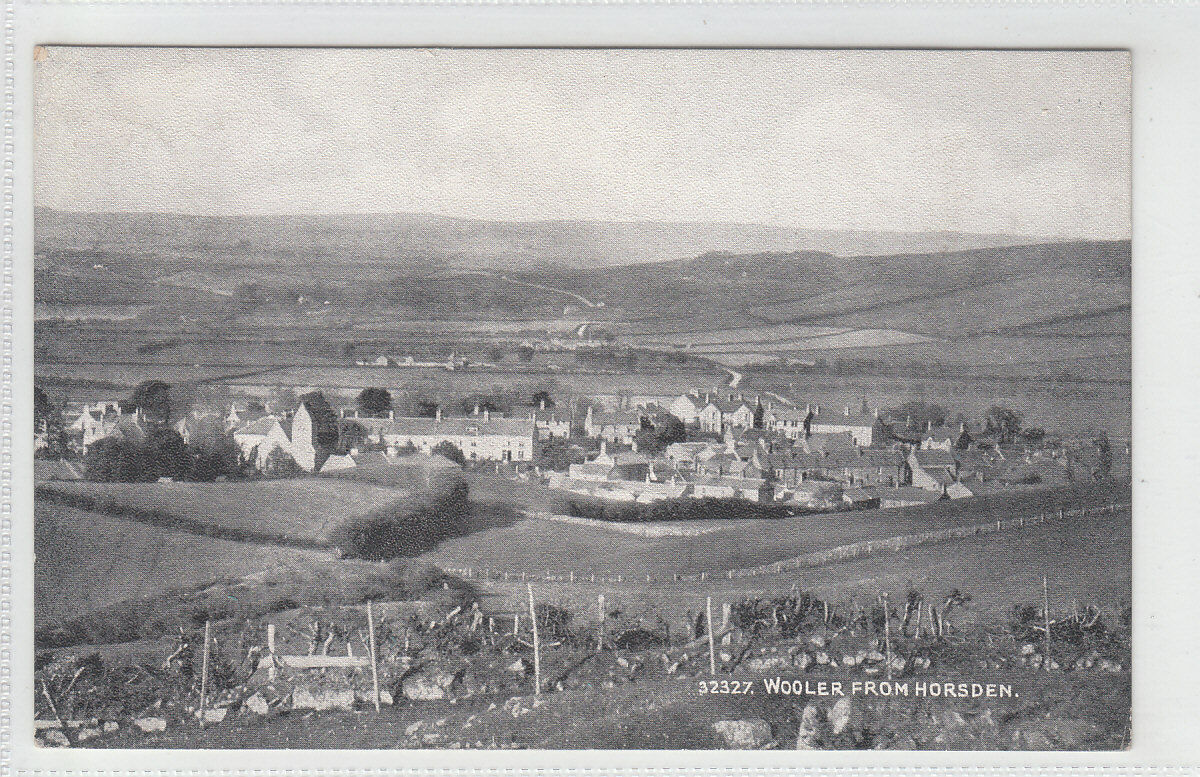This black and white photo, encased in a white frame with stitching around its leather-like borders, encapsulates a scenic countryside view with rich, historical depth. The image appears slightly aged, rendering the sky in varying grayscale tones. 

From an elevated vantage point, possibly a hill, the photograph looks down upon a pastoral town. The top quarter of the image is dominated by a grayish sky, leading into a horizon lined with slightly rolling hills and a blend of flat land. In the middle section, scattered houses and a prominent rectangular building, which could be an apartment complex or a university edifice, anchor the composition with their structured presence. Surrounding this central cluster are rocks, small trees, and signs of agricultural activity, hinting at a farming landscape. 

In the foreground, a rocky terrain presents itself, dotted with vertical wooden posts that resemble remains of a wire fence, hinting at past or ongoing land management. This section also features some dead trees and sparse vegetation, reflecting a possibly neglected or transitional area. 

Printed at the bottom right corner in white, the text "327 Wooler from Horsden" (or similarly rendered variations) adds a cryptic yet significant marker to the scene.